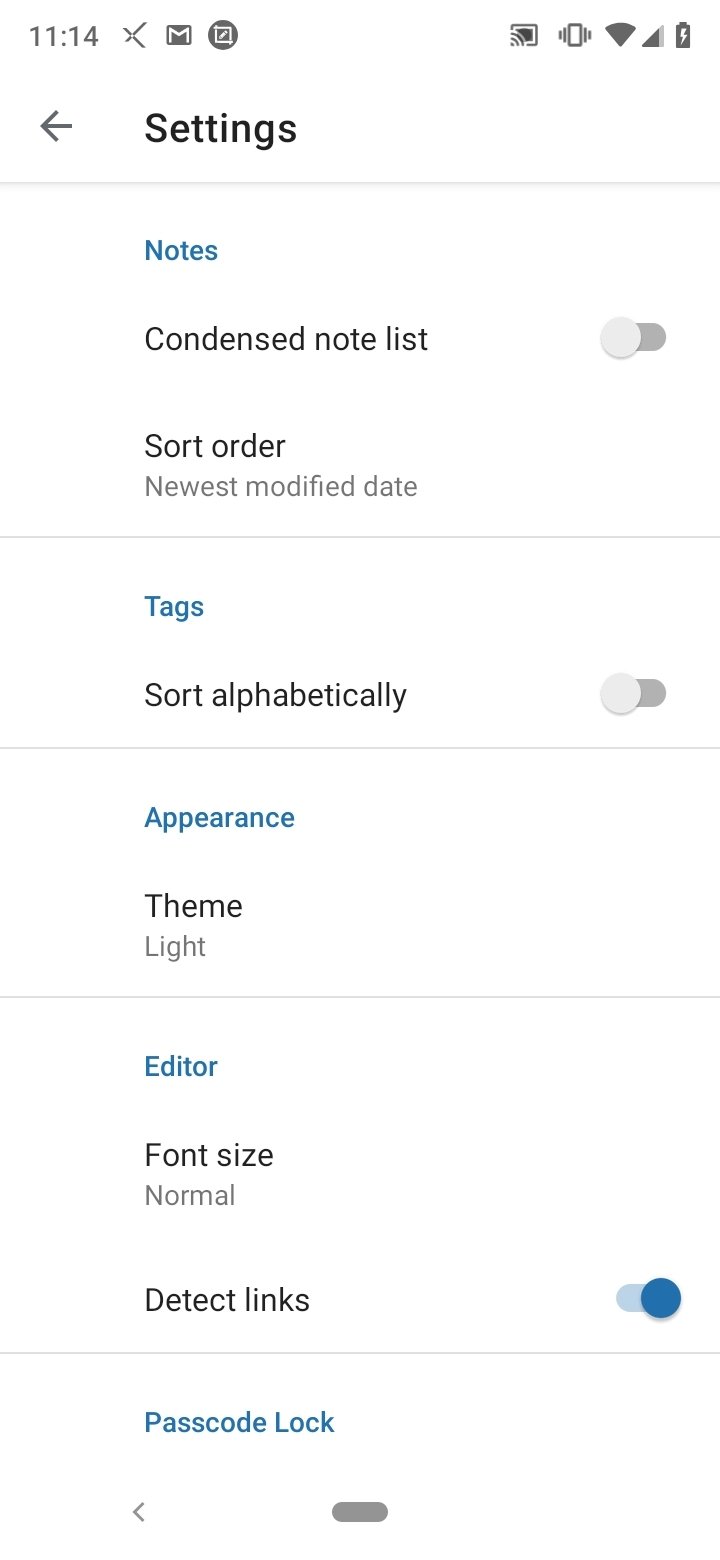The image displays a settings page with a predominantly white background and dark-colored text. At the top of the page, the time is shown alongside icons for Wi-Fi and battery percentage. The word "Settings" is prominently displayed in black text, accompanied by a grey back arrow to navigate back to the previous page.

Underneath "Settings," the word "Notes" is highlighted in blue text. Below this, "Condensed Note List" is written in black text with a grey switch indicating that the feature is turned off. The "Sort Order" setting follows, specified as "Newest Modified Date."

Next, the section titled "Tags" appears in blue text, and under this heading, "Sort Alphabetically" is written in black text with a grey indicator, showing that this feature is also turned off.

Further down, under the "Appearance" section, the "Theme" option is available, with the word "Light" shown in grey text. The next section, labeled "Editor" in blue text, includes a setting for "Font Size," which is set to "Normal" as indicated in grey text. The "Detect Links" setting, shown with a blue indicator, is turned on.

An option for "Passcode Lock" is also listed. At the bottom of the page, there is a grey back arrow with a small grey line beneath it.

Throughout the settings page, various interactive elements, such as buttons and switches, are used to toggle different features.